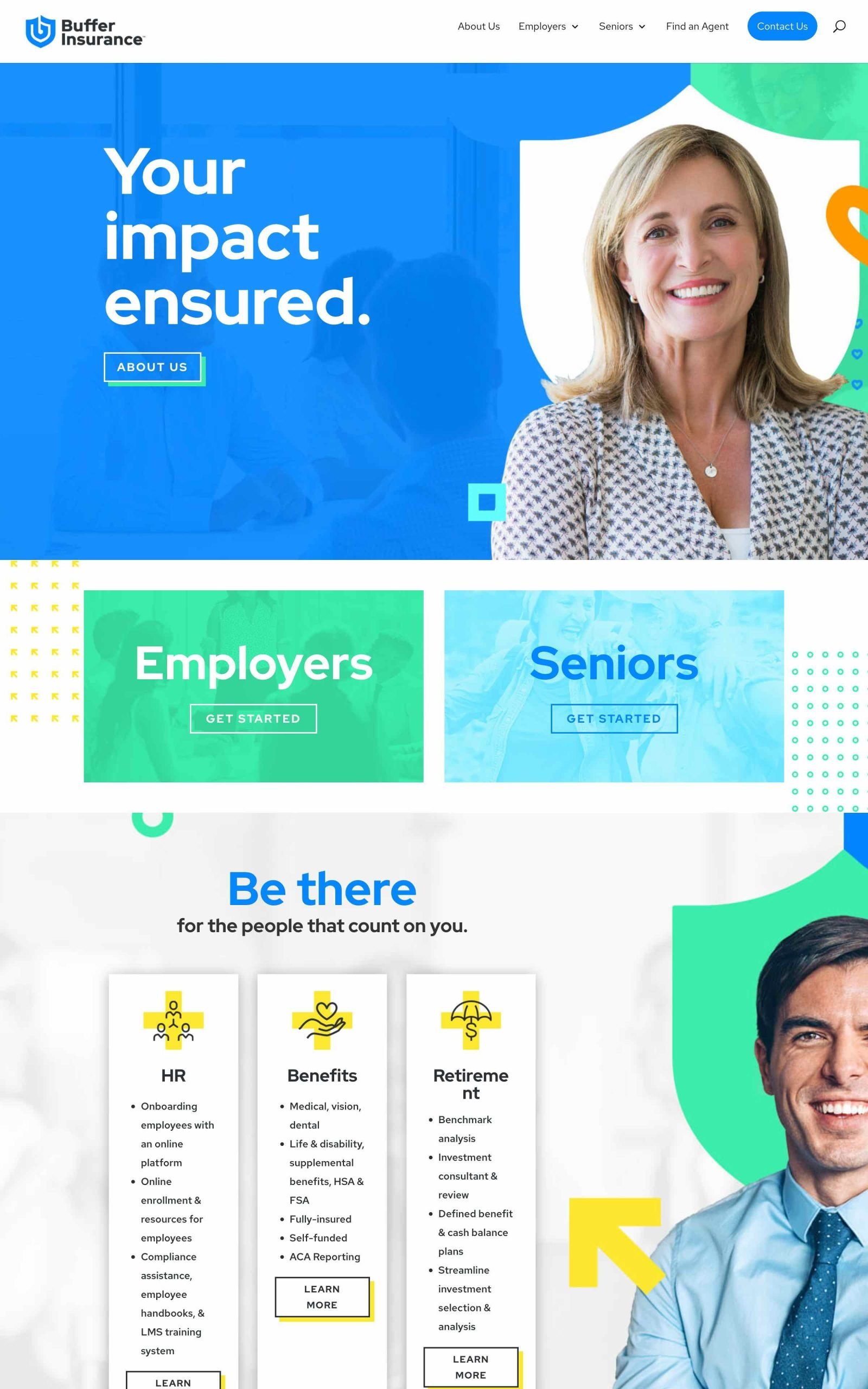The webpage for Buffer Insurance features a clean and professional design primarily with whites and grays. At the top, a prominent image with a blue background emphasizes the message "Your Impact Insured." Below, there’s a link to the "About Us" section showcasing a smiling woman in her 50s or 60s against a simple digital image of a white shield. The page also highlights sections for "Employers" and "Seniors" with prominent "Get Started" buttons. Further down, a motivating statement encourages viewers to "Be there for the people that you care about, be there for the people that count on you,” accompanied by an image of a smiling man in a business shirt and tie. The site also features sections on HR benefits and retirement, the latter marked with an added arrow for emphasis.